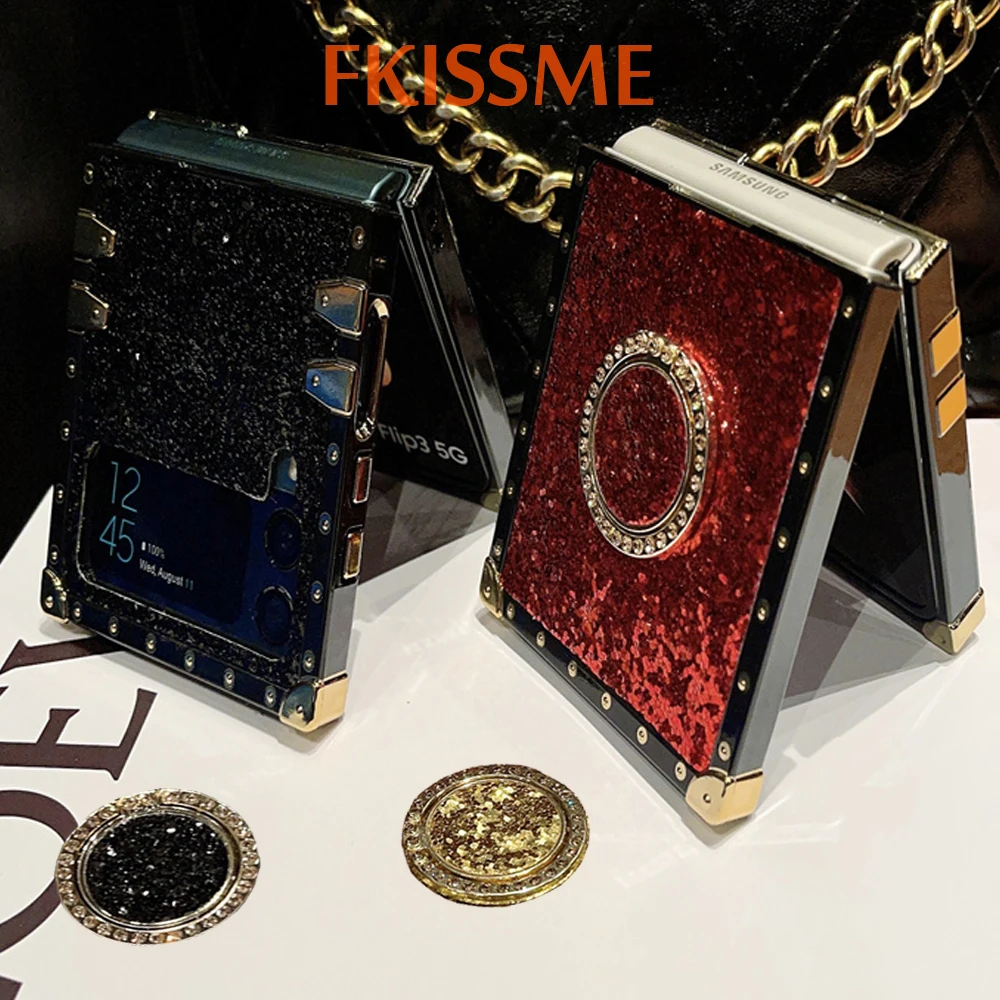The image depicts an advertisement for decorative phone cases designed for Samsung flip phones, with a brand title "Kiss Me" prominently displayed. Centered in the scene are two Samsung flip phones showcased with ornate cases. The phone on the right features a striking red case embellished with glitter and a circular arrangement of faux diamonds, resembling a jeweled accessory. To its left stands a sleek black phone case, accented with gold and sparkling details reminiscent of a starry night. 

In the foreground, placed on a white tabletop, are two circular pop socket-like accessories; the one on the left is black adorned with diamonds, while the right one glistens with gold and diamond-like accents. Above these items, a black patent leather purse with a gold chain handle complements the luxurious theme of the display. Embedded within the composition, the clock on one of the phones reads 12:45, adding a touch of everyday realism to the scene.